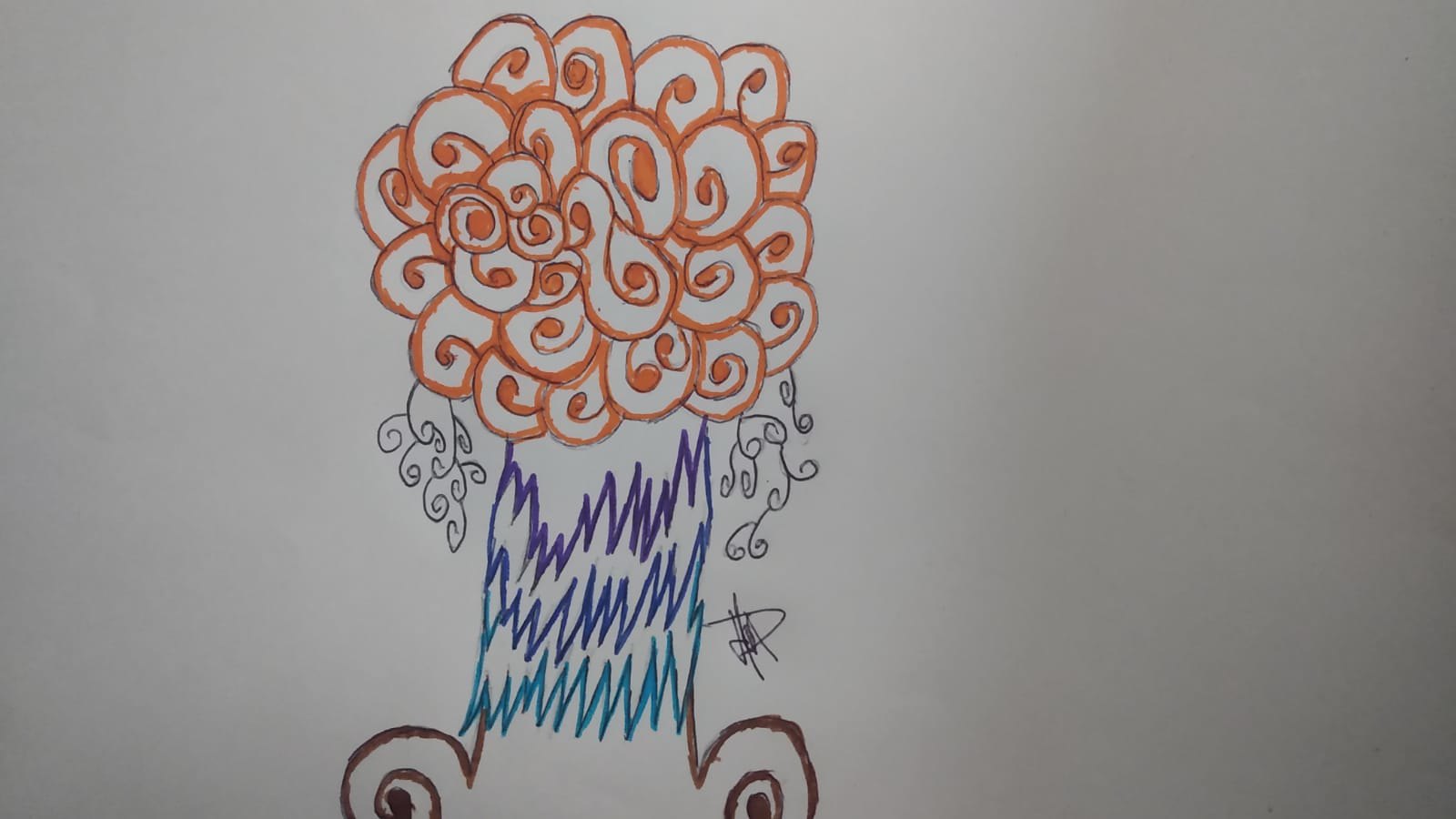This image is a horizontally cropped color photograph of a child's artistic drawing, prominently positioned against a grayish-white background. The drawing features a whimsical tree, showcasing a colorful and imaginative style. The tree's trunk is adorned with alternating zigzag patterns in light blue, dark blue, and purple. Emerging from the base of the trunk are two spiral shapes, resembling feet, colored in a rich brown hue and extending to the left and right.

The tree's canopy is intricately designed with tight curls, predominantly white in the center with an orange border encircling it. From the central portion, delicate vine-like tendrils and swirls, resembling leaves, extend outward to the left and right. These details are meticulously sketched in black ballpoint pen. The artist has signed their creation in black ballpoint pen, placing the signature just beneath the vine elements on the right side.